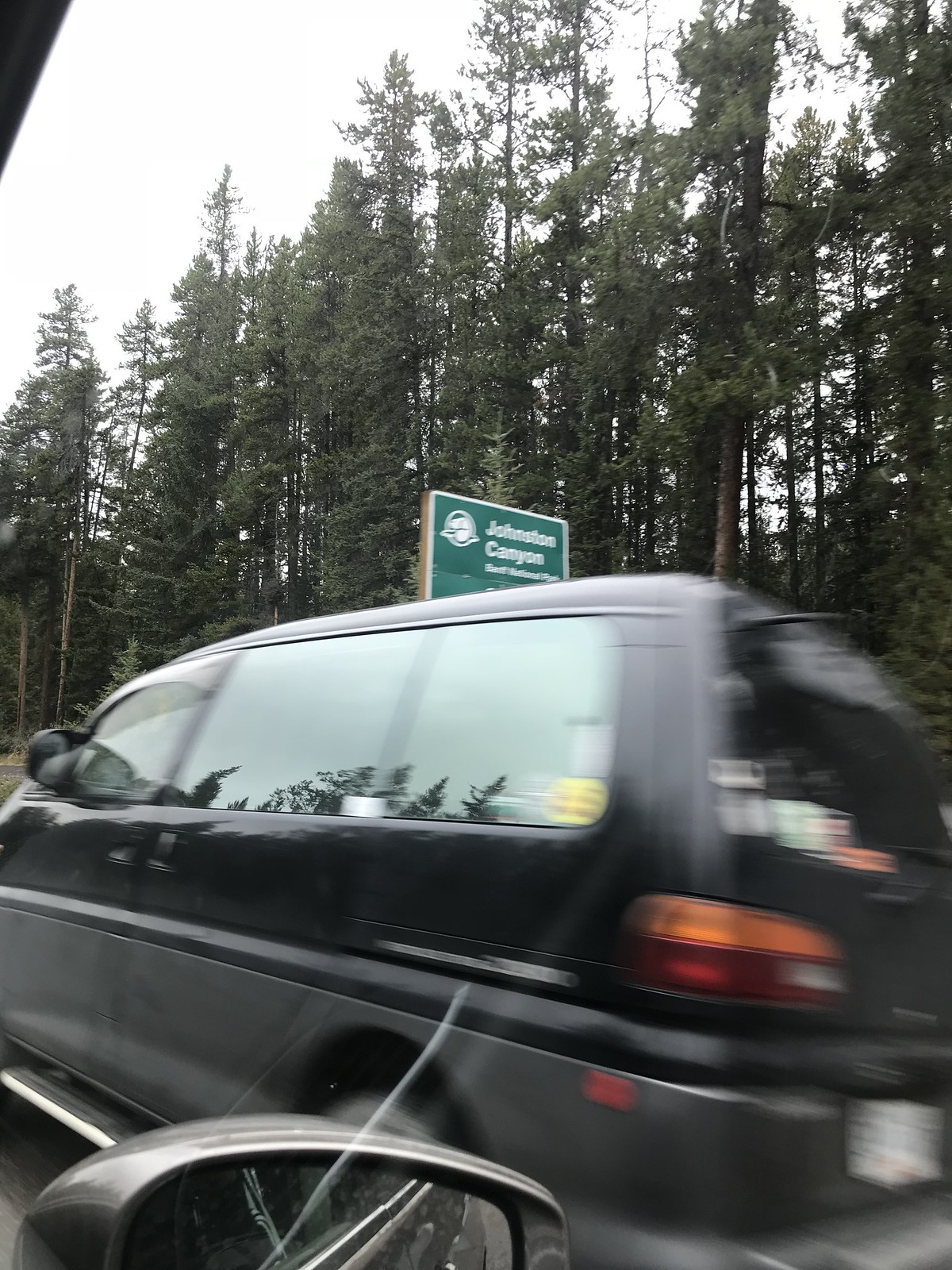The photograph captures a dynamic moment on the road as a minivan speeds past a car. The image is taken through the passenger window of the car, offering a slightly blurred view, indicative of the fast movement. The minivan, adorned with various stickers on its rear, features distinctive red and orange taillights, a white license plate that is not clearly visible, black trim, and gray sideboards designed for easy step-up access.

In the background, there is a green road sign bordered in white, partially readable, suggesting destinations like Johnston Canyon, Black National Park, or possibly Banff National Park—though the exact wording is indeterminate. The top left corner of the sign is marked with a green leaf-like emblem that adds a touch of character.

Encasing the scene is a lush backdrop of tall, slender evergreen trees with pointed tops, contributing to the natural ambiance. In the foreground, the side mirror of the car from which the picture is taken is just visible, grounding the viewer in the current vehicle's perspective.